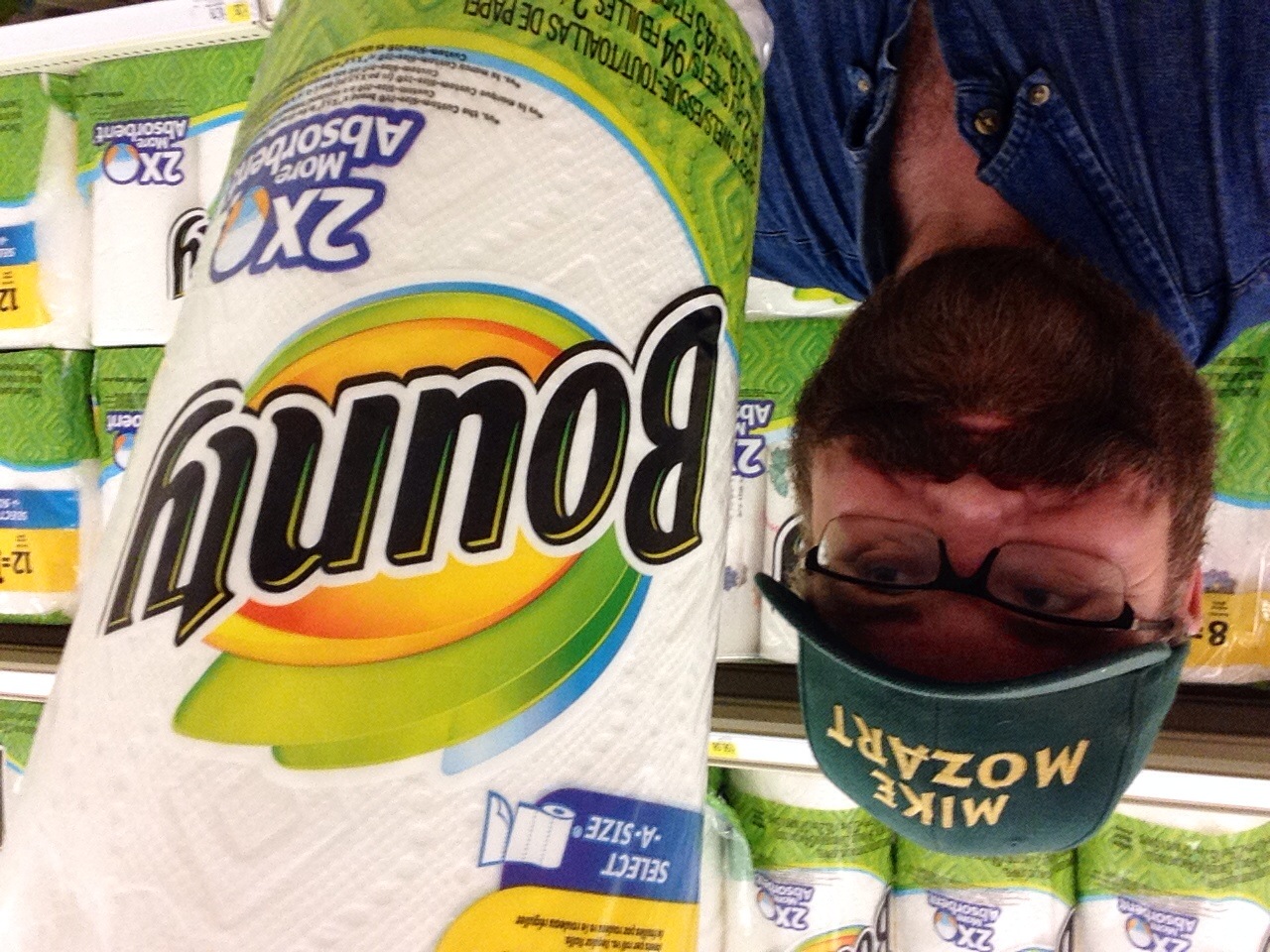In this photograph, a fair-skinned man with rosy cheeks is standing in a store, posing in front of a shelf lined with stacks of Bounty paper towels. He is wearing a green hat with "Mike Mozart" written in red letters, black-frame glasses, and a blue, slightly shiny button-up shirt, with the top two buttons unbuttoned. His thick, well-lined beard and mustache frame his face, which sports a cheesy smile. He holds a roll of Bounty paper towels, still in its plastic wrap, and looks at it lovingly. The roll features bold black letters reading "Bounty" with a white outline. The packaging is designed with a gradient swirl pattern in yellow, green, and blue, and prominently states "two times more absorbent." The man, identified by his hat, and the colorful, neatly displayed paper towels create a cheerful and vibrant scene.